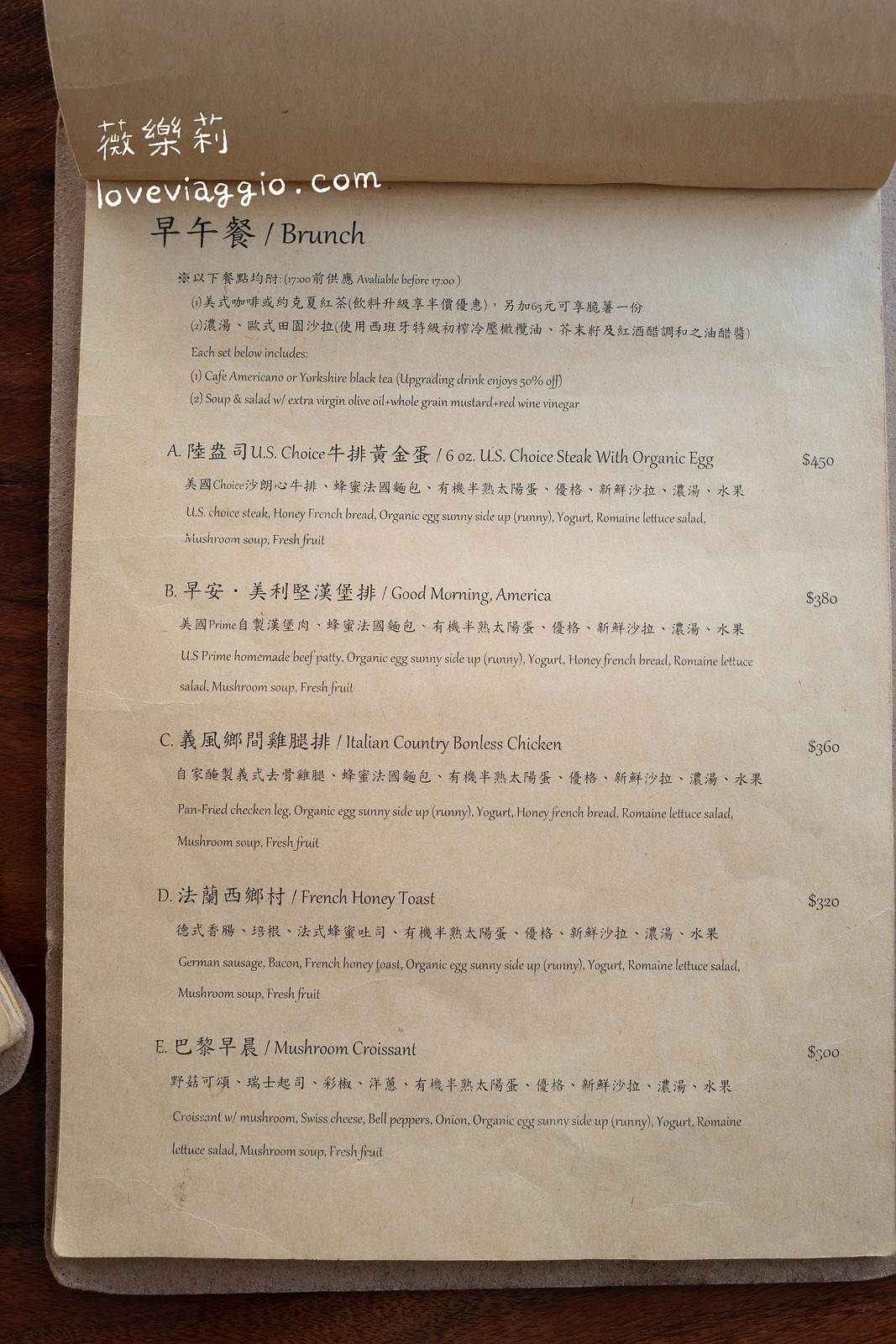This vertical image depicts a page from a restaurant menu in exquisite detail. In the upper left corner, an overlay features Asian characters, possibly denoting the restaurant's name or a thematic element. Below this, the website "loveviagio.com" is prominently displayed, suggesting that the restaurant is named Viagio. The menu page itself has a parchment-like quality, reminiscent of tan, aged paper. The text, inscribed in elegant black ink, is small and intricate, blending Asian characters with English descriptions.

The menu items include an intriguing array of dishes. At the top, a six-ounce U.S. Choice steak paired with an organic egg is priced at $4.50. Following that is an offering named "Good Morning America," described as a type of breakfast yogurt, priced ambiguously at either $8.38 or ¥8,380, indicating the possibility of a price listed in yen. Next, "Italian Country Boneless Chicken" is presented as a savory option. The final items on this eclectic menu are "French Honey Toast" and a "Mushroom Croissant," rounding out a diverse and international selection of dishes.